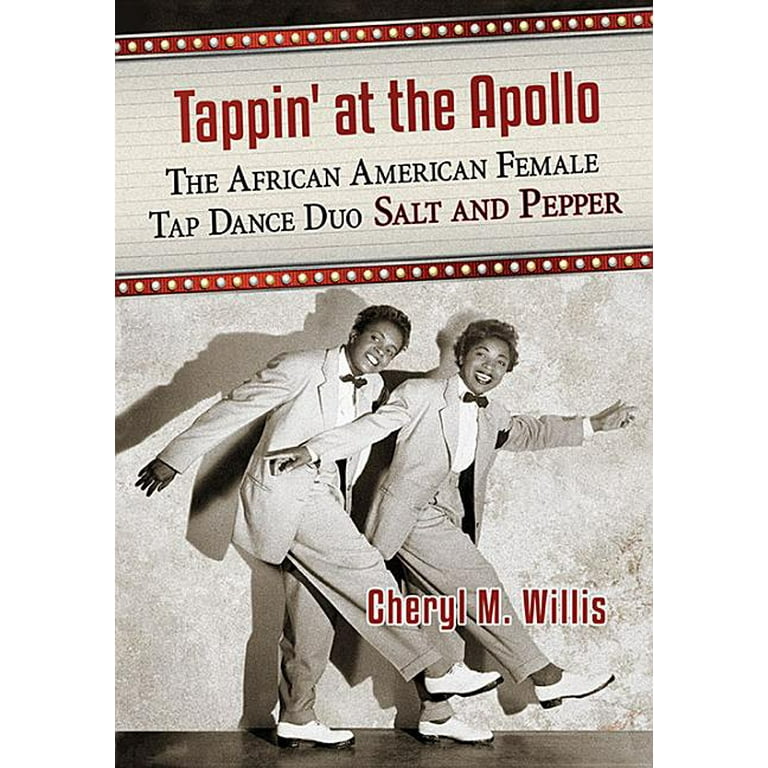The book cover for "Tapping at the Apollo" features a vintage-style black and white photograph of the renowned African-American female tap dance duo, Salt and Pepper. The title, "Tapping at the Apollo," appears prominently in bold burgundy letters at the top, followed by the subtitle in black lettering: "The African-American female tap dance duo Salt and Pepper." Below this text, a quick line of alternating white and yellow marquee lights over a red strip adds to the vintage aesthetic.

The photograph captures Salt and Pepper in the midst of a dynamic tap dance routine. Both women, with short hair and expressive, bold lipstick, are adorned in black tuxedos complete with bow ties and wide-legged trousers. They wear white tap shoes with black heels. Positioned in remarkable synchronization, both dancers have their right leg set apart and their arms outstretched, poised and smiling brightly as they engage with their audience. The dark wood floor beneath them is contrasted by subtle shadows that enhance the depth of the image.

In the lower right corner of the cover, the author's name, Cheryl M. Willis, is elegantly printed in burgundy letters, cementing the connection between the vibrant visuals and the storytelling within this captivating book.